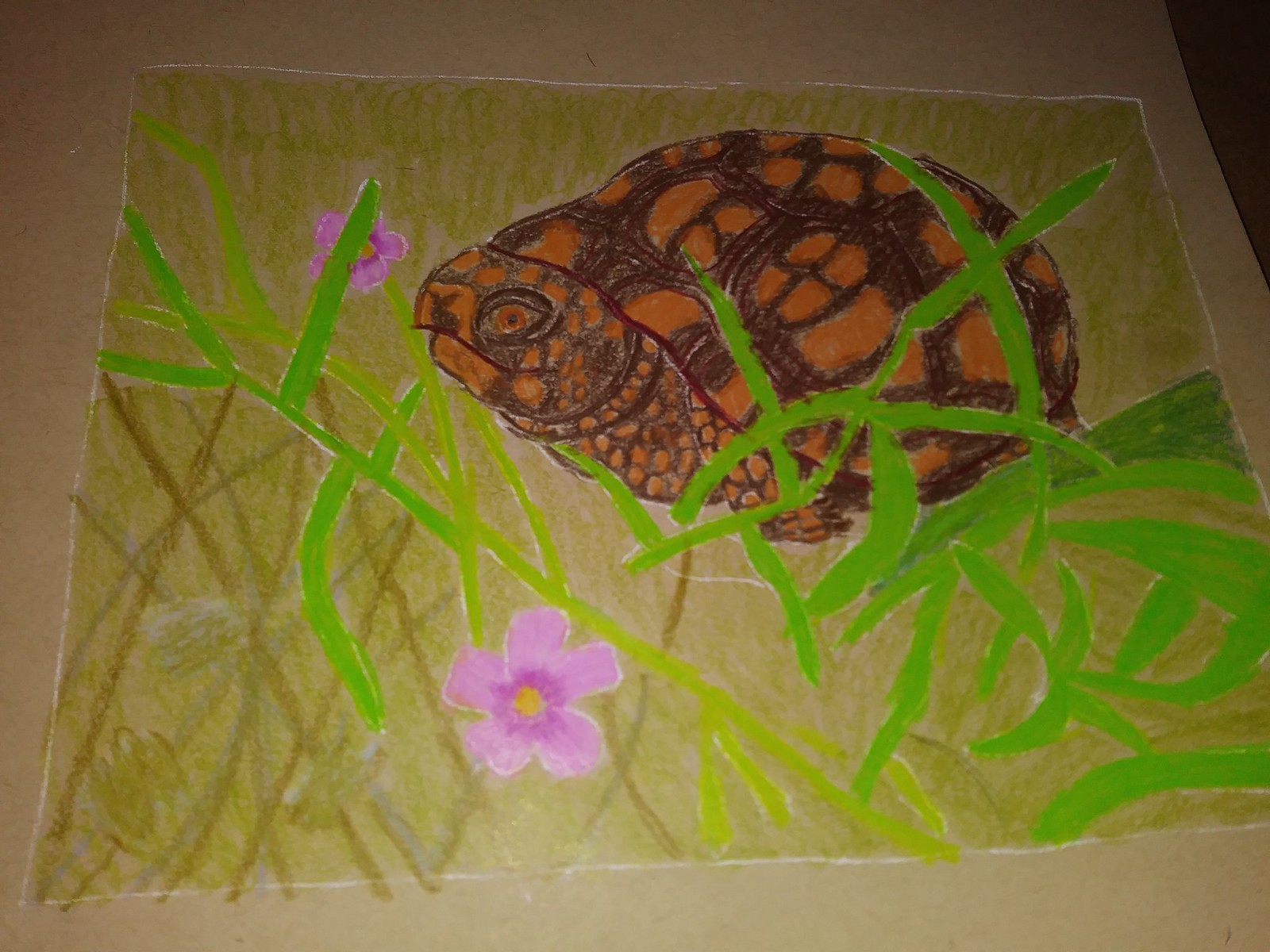This is a photograph of a child's detailed drawing, possibly colored with crayon, marker, or watercolor, on a piece of white or construction paper laying on a light brown table. The artwork features a realistic and detailed turtle, prominently occupying the center of the image, about 50% of the drawing. The turtle is depicted in vibrant shades of orange and black, with intricate scale patterns and scoring lines on its shell. Its head, adorned with orange eyes, is poking out while its feet are tucked under its body.

The turtle is surrounded by a lush, multi-colored grassy field. The grass blades vary in shades including pea green, bright green, lime green, dark green, and even some lighter greens, with elements of yellow and brown mixed in. Among the grass, there are two prominent pink flowers, one purple with a yellow center and another pinkish-purple one partially obscured by grass. The scene captures a vivid and lively habitat, emphasizing the turtle's natural surroundings in a vibrant and engaging manner.